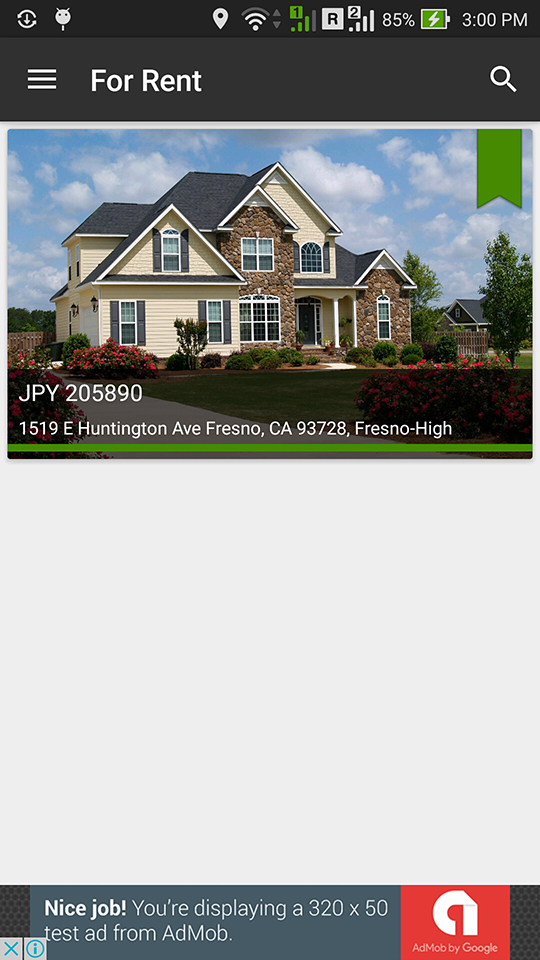The image is a screenshot from a cell phone or tablet showcasing a house available for rent. At the top, a prominent banner in large white letters reads "For Rent," accompanied by three horizontal bars and a magnifying glass icon, suggesting a search function. 

The house itself is a striking two-story building, characterized by a mix of white siding and stone-faced exterior. The front facade features four distinct gables, with additional peaks visible on the sides, contributing to its dynamic roofline. A series of double-hung rectangular windows punctuates the front, including a large picture window with numerous small panes.

The entryway, located on the right third of the house, is accessible via a set of stairs. The landscaping is meticulously maintained, with a broad swath of pink flowers on the left side of the building, a small bush or tree between some windows, and shorter shrubbery flanking the stairs and wrapping around the right side.

Around the corner from the main entrance, the left side of the house reveals a garage, illuminated by lights on either side and featuring a side entrance door. A paved driveway leads up to this area.

Beneath the image, the text "JPY 205890" is displayed, followed by the address: "1519 East Huntington Avenue, Fresno, California, 93728." The location is further identified as "Fresno High."